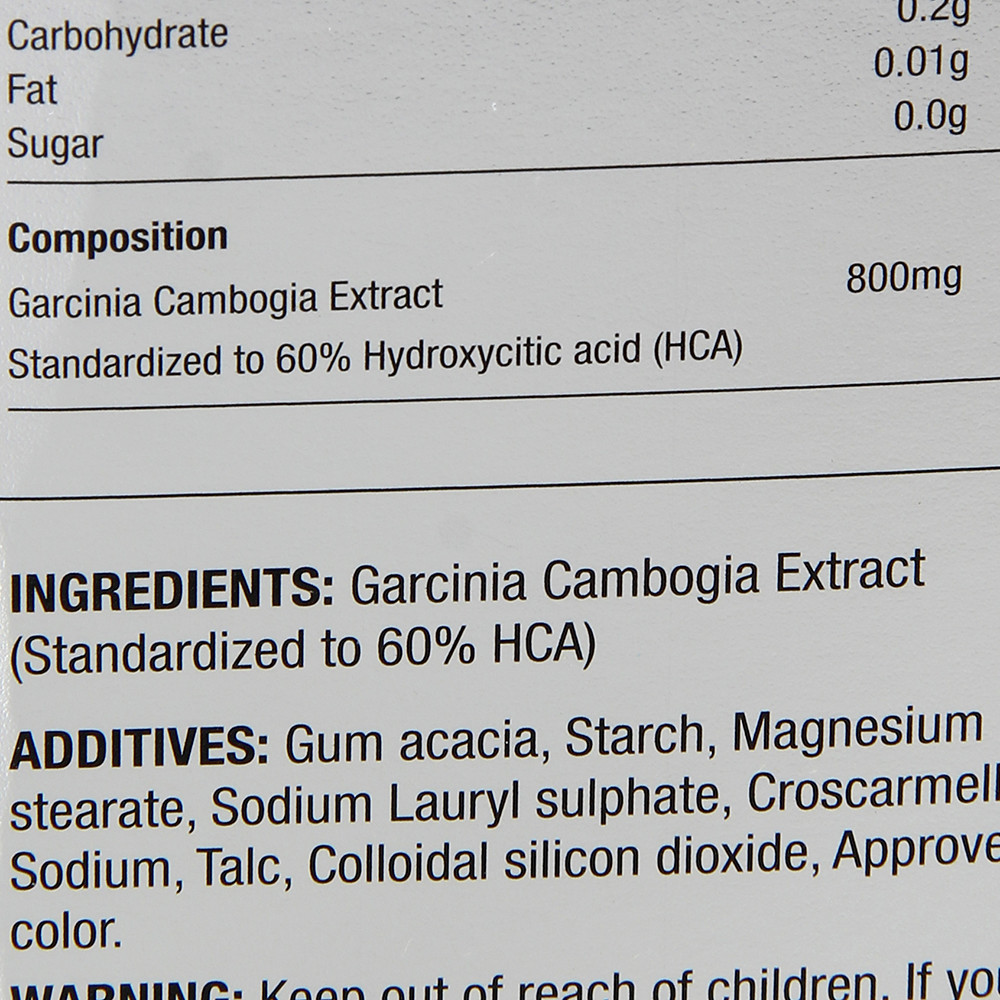A highly zoomed-in, close-up view of a nutritional label on the back of a food product. The top part of the label, where it presumably says "Nutritional Facts," is not visible, and some of the text is cut off due to the extreme zoom. The label has a gray background with black lettering. It lists the following nutritional information and ingredients:

- Carbohydrates: 0.2 grams
- Fat: 0.01 grams
- Sugar: 0 grams
- Garcinia Cambogia Extract: 80 milligrams, standardized to 60% Hydroxycitric Acid (HCA)

Ingredients include:
- Garcinia Cambogia Extract, standardized to 60% HCA
- Additives: Gum Arabic, Asparagus Starch, Magnesium Stearate, Sodium Lauryl Sulfate, Sodium Alginate, Colloidal Silicon Dioxide, and approved colorants.

A portion of a warning is visible, advising to keep the product out of reach of children, though much of the warning is obscured by the bottom and right edges of the image.